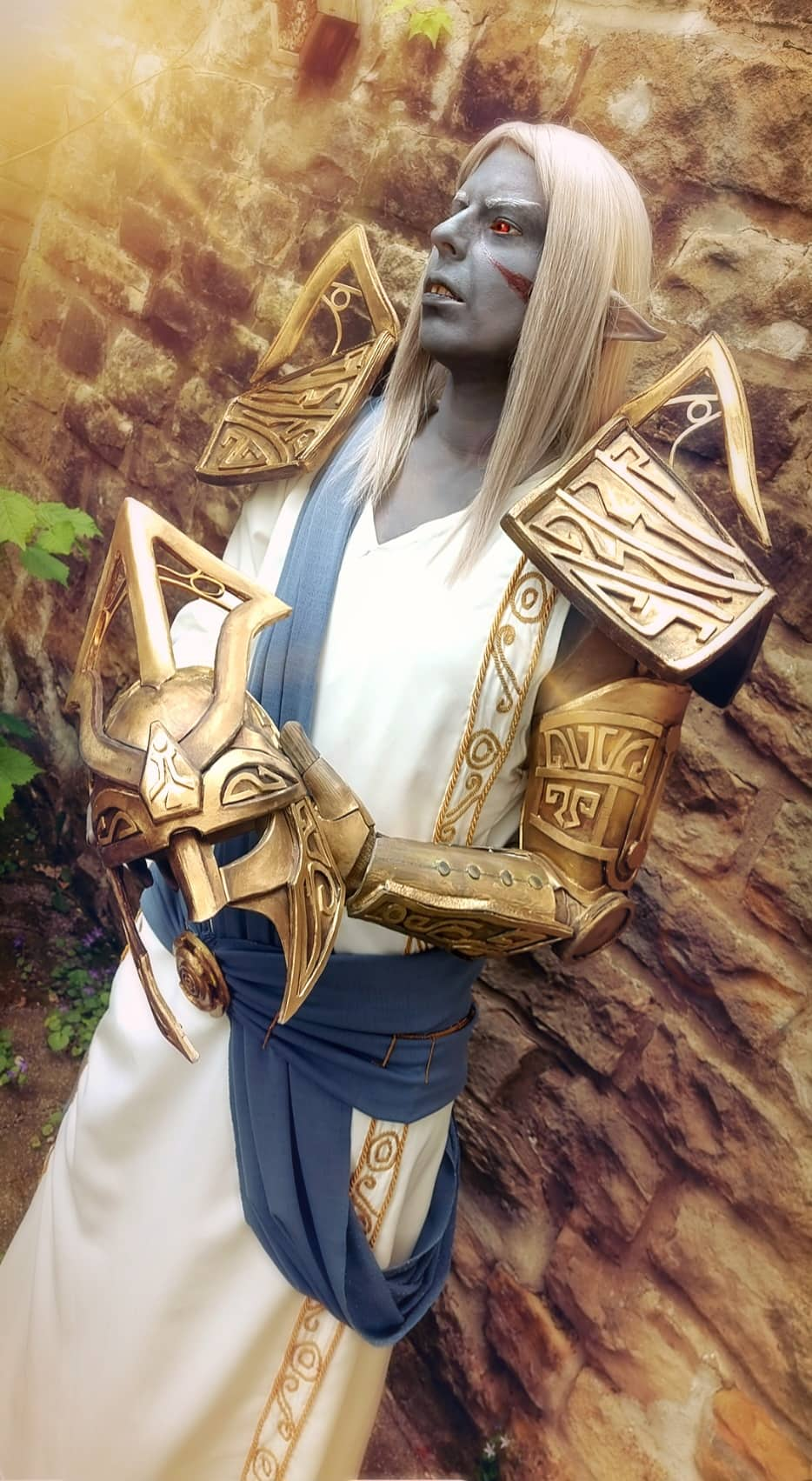In front of a brown stone wall, a highly detailed, computer-generated image depicts a character from the game Elder Scrolls, specifically Sotha Sil. The character has striking, long creamy brown hair cascading past his shoulders, blending into his intricate gold armor. His skin is pale grey with distinctive red triangular markings on his cheeks, and his eyes are a piercing red, accented by white eyebrows. Tall, pointed elf ears emerge from his hair, contributing to his otherworldly appearance.

The character's attire includes a long, elegant white gown with a V-shaped collar, adorned with gold scrollwork down the side and a blue sash draped around his waist and shoulder. On his right arm, he wears detailed golden armor. Over his shoulders sits a brown metal seal with a random pattern and a prominent triangular shape on top, giving him a regal appearance.

In his hands, he holds a bronze helmet featuring a shield-like design that would cover the eyes and part of the face. The helmet bears a striking resemblance to a ceremonial or protective piece. Sotha Sil's gaze is directed toward the left, as if looking into the distance. The scene is accented with hints of greenery, suggesting the presence of trees or plants near the stone wall, further enhancing the lifelike realism of the image.